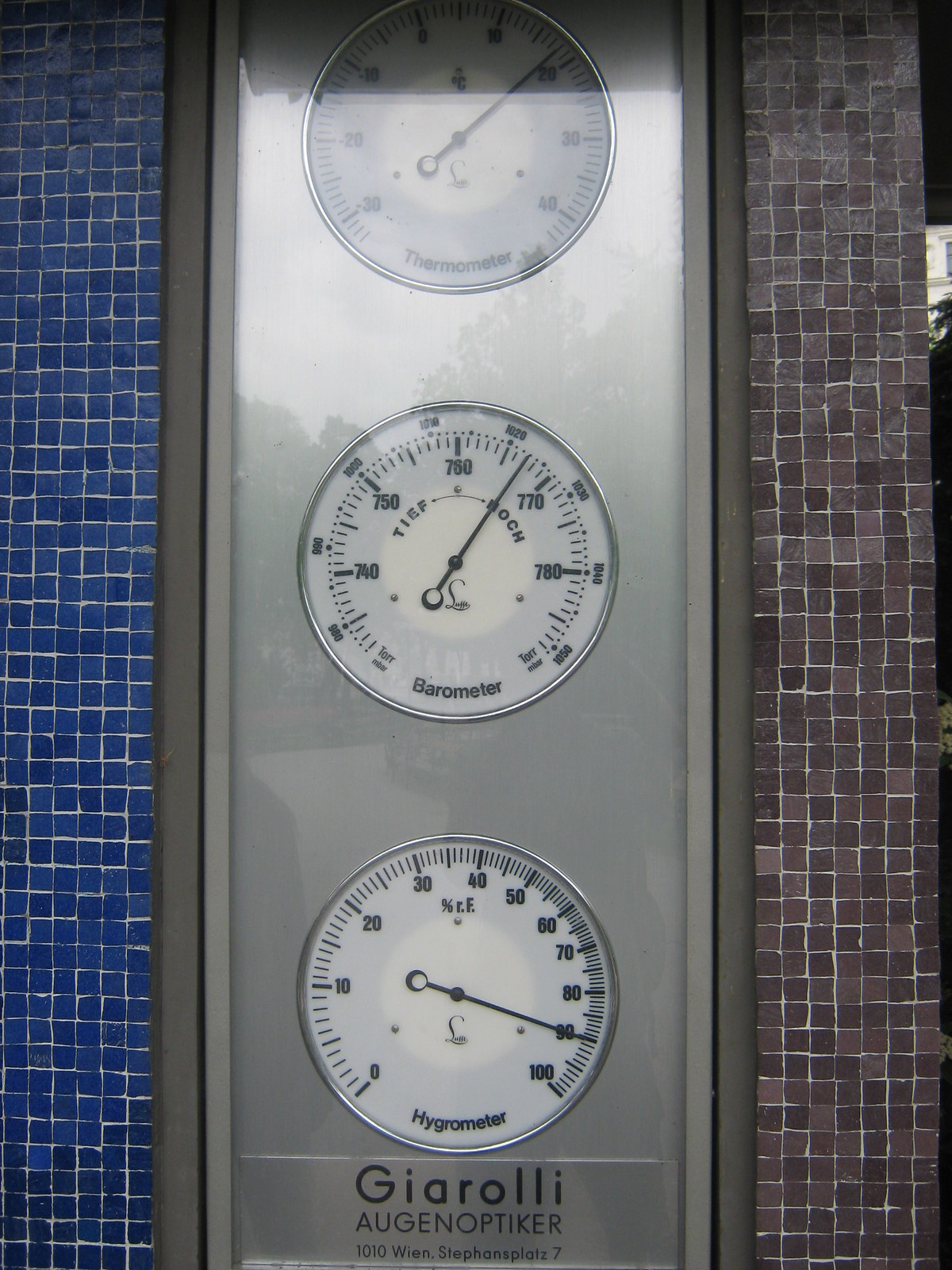The image showcases a rectangular, vertically mounted, metal instrument panel inset with three circular dials. The panel is bordered with a darker grey trim and has a recessed edge, giving it a sophisticated appearance. Each dial features black handles and black text on white backgrounds. The top dial is a thermometer, marked in Celsius, with the needle pointing to just under 20 degrees Celsius. The middle dial is a barometer, indicating a barometric pressure of approximately 767 (units not specified). The bottom dial is a hygrometer, displaying a relative humidity of 90%. Beneath these instruments, there is a label that reads "Giroli-Augenoptiker, 1010 Wien, Stephansplatz 7," suggesting a German or Austrian origin. The panel is mounted on a wall with small, blue square tiles to the left and reddish-brown tiles of a similar size to the right, both with grey grout. This detailed setup provides a thorough and clear depiction of the various environmental measurements.